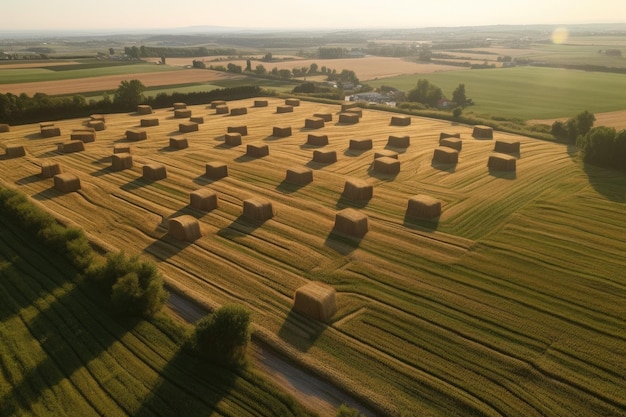In this outdoor daytime photograph, we're greeted by a serene agricultural landscape dominated by neatly arranged bales of hay. The foreground captures a close-up of a field with approximately 40 large, compact square bales. These substantial blocks of hay, almost large enough to fill a pickup truck bed, are laid out in several orderly rows. Adjacent to this hay field on the left runs a dirt road flanked by a row of trees, while a gentle stream meanders nearby.

To the right of the hay bales lies an expansive green field, bearing the subtle tracks of recent tractor activity. Behind this, a large house punctuates the rural scene. The rolling plains stretch outwards, revealing a harmonious mix of light beige and golden hues, the result of harvested hay. The terrain is mostly flat with gentle bumps rather than steep hills.

In the background, the sky is bathed in a warm, buttery yellow tone, suggesting either morning or late afternoon sun. The sun itself, a circular orb, shines from the top right corner, casting a pleasant glow over the entire landscape. Additional trees can be spotted both in the foreground on the left and scattered in the more distant parts of the scene, framing this picturesque and tranquil setting.